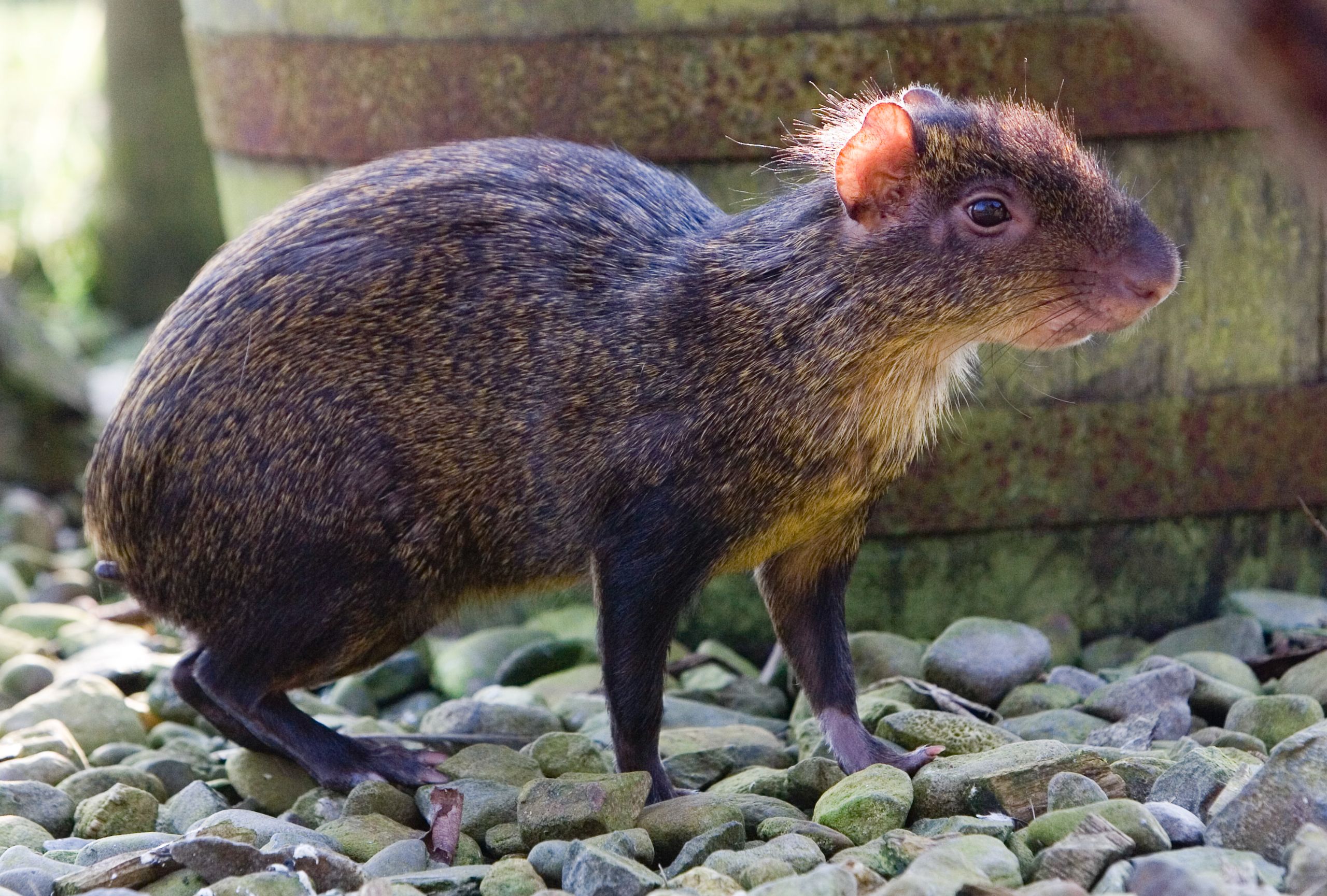This is an image of a small rodent-like animal, possibly a young muskrat, chipmunk, or a different type of rodent, featuring a combination of traits from all suggested animals. The animal has a light brown fur coat with black spots and a calico pattern, and its long hind legs support a hump in its back. It has small, slightly pinkish ears that poke above its head, almond-like eyes, and long, claw-like nails. The animal is standing on a mixture of gravel and small gray rocks. In the background, there is a blurry scenery with foliage and hints of sky, alongside a rusted gray wall with horizontal orangish-brown rust stripes resembling a garden barrel. The rodent takes up most of the picture and is facing to the right of the viewer.